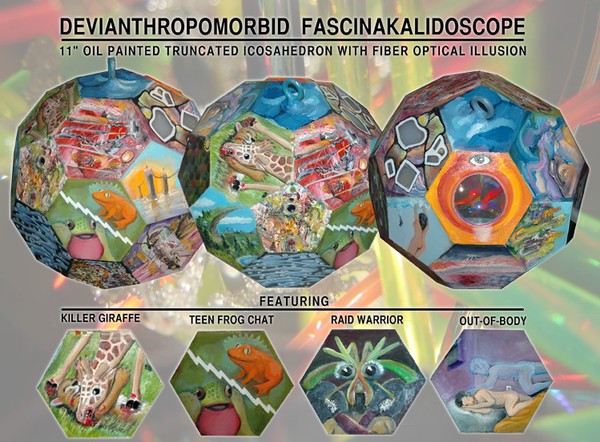The image presents a vivid and detailed depiction of geometric artwork, with a clear mix of animals and abstract designs. At the top, black text reads "Deviant Thropomorbid Fascinakaleidoscope," with the latter term underlined. Below this title, a smaller caption states: "11-inch oil-painted, truncated icosahedron with fiber optical illusion."

The central section showcases three large, roughly 10-sided geometric shapes, overlapping slightly. Each is a riot of colors – orange, blue, pink, brown, and gray. The left shape prominently features an orange frog, the middle reveals a spotted giraffe at its center, and the right displays a hexagonal design in shades of orange and red, with an eyeball at the top.

Beneath these shapes, the underlined word "FEATURING" introduces four smaller hexagonal images. From left to right, they include: a "Killer Giraffe" with a blood-stained appearance, a "Teen Frog Chat" showing two frogs (one orange, one green), a "Raid Warrior" with a creature sporting long ears, two eyes, and horns, and an "Out of Body" scene depicting a naked person lying on a bed with a spirit-like form hovering above.

The entire composition conveys a sense of vivid artistic exploration and complex design, all encapsulated within a kaleidoscope-like theme.